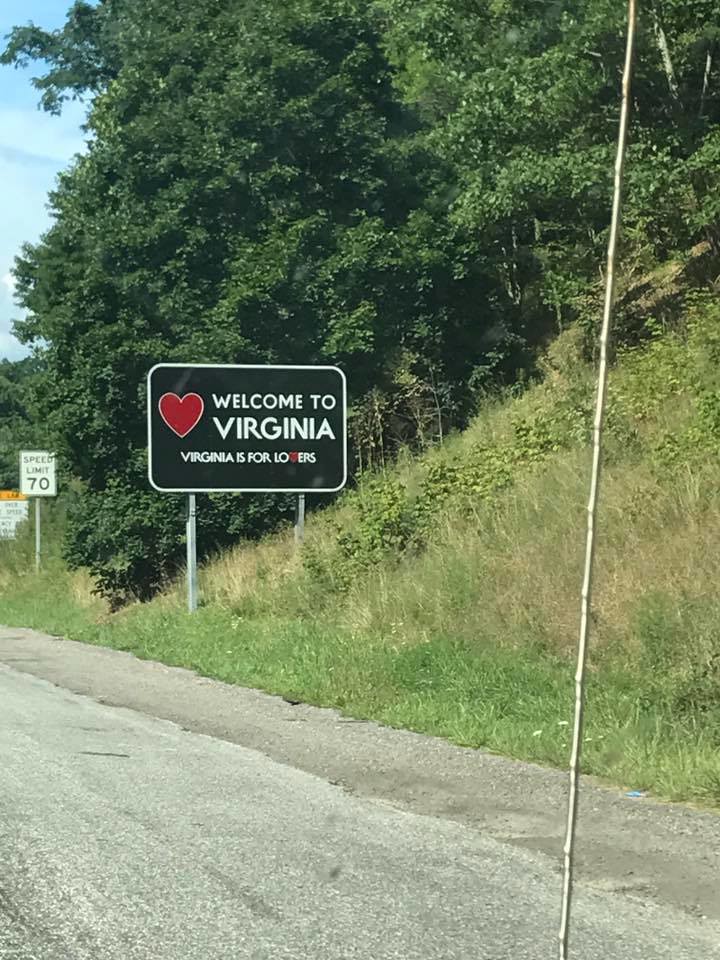The photograph captures a segment of a gray, paved highway that curves off to the right and appears slightly worn, indicating it's in need of repair. The road is edged by a darker brown-gray strip, with a lush, green grassy hillside rising on the right, leading to a dense stand of full, verdant trees. Dominating the scene is a prominent black rectangular sign on metal posts, displaying the white-lettered text, "Welcome to Virginia. Virginia is for lovers," with a large red heart outlined in white beside the text. The 'V' in "Virginia" is also red. Just beyond this, a smaller white rectangular sign reads, "Speed Limit 70." The sky in the upper left corner of the photo is a bright blue with a few stray clouds.